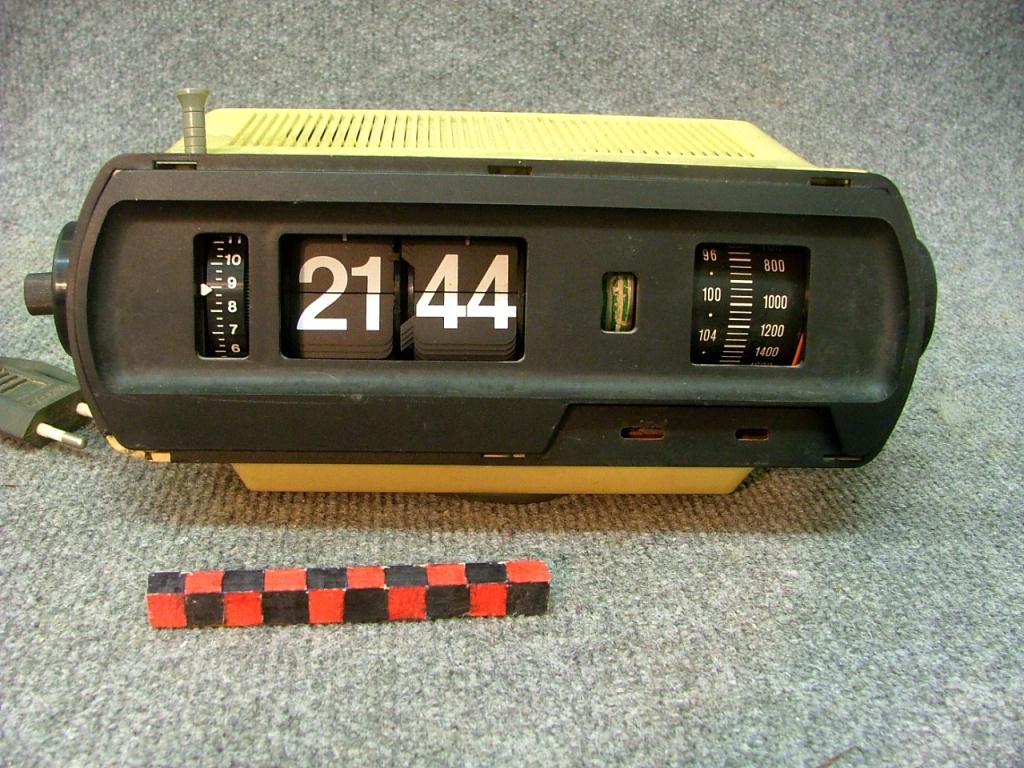This photograph depicts a vintage flip clock radio placed on a gray carpet. The device is rectangular with a yellow body featuring vent-like cuts at the top. Its face, framed in black, prominently displays an old-fashioned flip clock mechanism showing the number 2144, suggesting it might not be a traditional clock. The clock's face includes two rectangular areas: the left side houses a vertical dial with numbers 10-9-8-7-6 and a small white arrow, indicative of a tuning function. The right side contains a wider dial with ranges from 96 to 104 on the left and 800 to 1400 on the right, hinting at AM-FM radio capabilities. A black plastic plug is visible on the left side of the clock. In front of the clock lies a rectangular stick or piece of wood painted with a red and black checkerboard pattern.